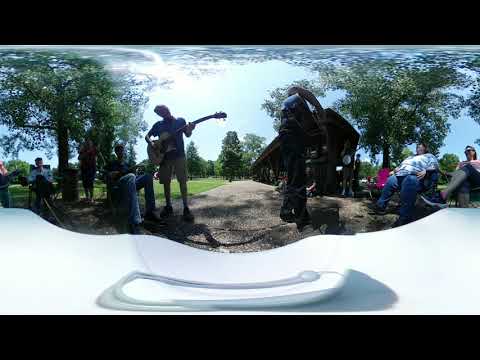The photograph captures an outdoor scene in a park or wooded area with a slightly distorted, panoramic view. Central to the image are two musicians, one on the left wearing a blue t-shirt, cargo shorts, and hiking boots, playing an acoustic guitar while seated on a cobblestone walkway. To his right, another person is also playing the guitar, though his back is turned to the viewer and he appears to be wearing jeans. Both musicians are surrounded by an audience of people seated on either side, enjoying the music. The setting includes tall green trees under a vibrant blue sky, enhancing the natural ambiance. Additionally, there is an outdoor structure with a roof visible on the right, offering shade from the sun. A white object, possibly a table, is present at the front of the image, adding to the overall scene, with a black border on the top and bottom framing the photograph. Despite the slight blurriness and distortion, the sense of a communal, musical gathering in a serene, natural environment is well conveyed.